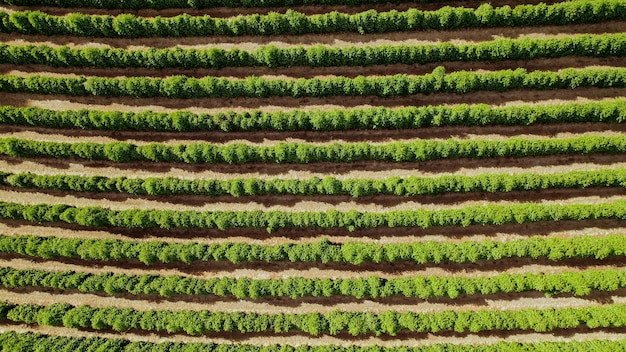This aerial color photograph, taken outdoors during the daytime, captures a meticulously arranged farm landscape viewed from high above. The image, lacking a border and background, is a horizontally rectangular frame filled entirely with an array of horizontal rows of lush green plants or trees, tightly packed and dense. Between these verdant rows, visible strips of brown dirt create a repeating pattern that spans the entire width of the image from left to right. The shadows cast by the plants, influenced by the overhead sunlight, highlight the texture and layout of the farm. As the rows recede towards the top of the image, the ground appears darker, enhancing the depth and dimension. This repetitive sequence of green rows and brown dirt dominates the photograph, encapsulating the essence of well-ordered agricultural practice.